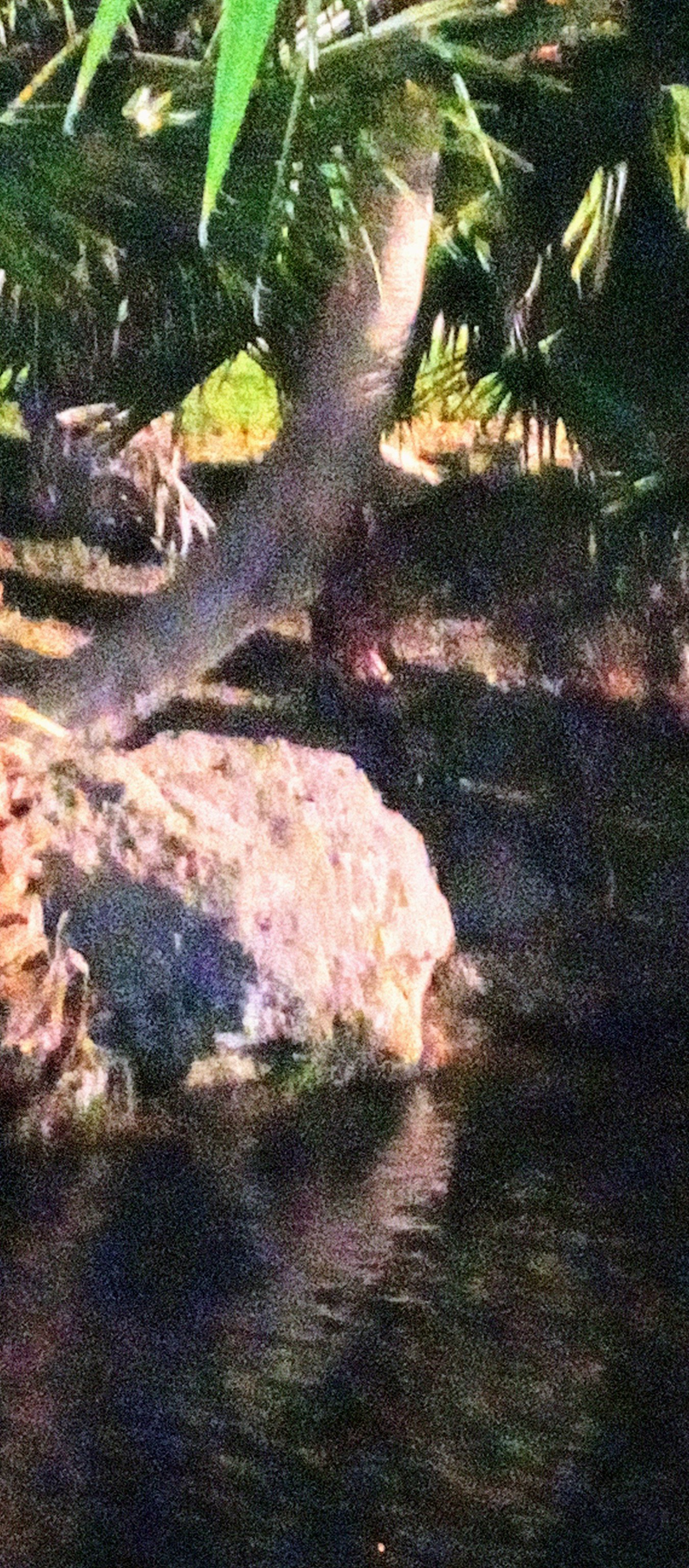This photograph, which appears grainy and of low resolution, depicts a serene natural scene in a vertical portrait orientation. At the top of the image, a riverbank is visible, partially covered with green grass and some brown soil. A distinctive plant, possibly a tree with a curving trunk, extends from the edge of the frame, displaying long, thin leaves that appear as angular fronds, suggestive of a palm tree. This trunk exhibits a brownish-grey color and creates a sense of depth, with some leaves arching down from the very top edge of the frame into the foreground.

Below the riverbank, a dark body of water spirals from the middle right towards the bottom left corner of the photograph, its surface faintly reflecting parts of the brown riverbank. The water, potentially a lagoon or a small pond, shows signs of green algae. Shadows from the plant or tree trunk add depth to the scene. Surrounding the water and extending into the background, rocks and patches of dirt add to the naturalistic environment, evoking imagery of a small, secluded garden oasis enveloped in abundant green foliage.